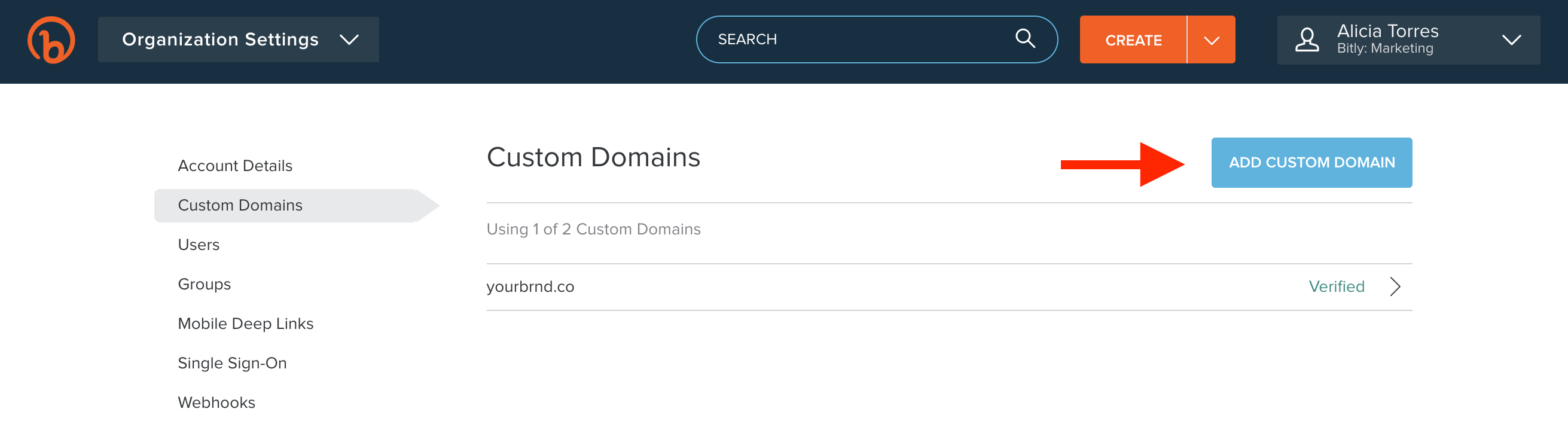The image appears to be a screenshot of an organizational management website. 

**Top Section:**
- **Top Left:** The logo of the site, which is an orange circle with a stylized letter 'B' inside it, is displayed. Next to the logo, within a boxed area, the words "Organization Settings" are visible, accompanied by a small downward-pointing arrow.
- **Top Center:** In the middle of the top section, there is a prominently displayed search bar. The left side of the search bar has the word "Search" in it, and the right side features a magnifying glass icon. The search bar is currently empty.
- **Top Right:** To the right of the search bar, there is an orange rectangular button with the word "Create" inside it, along with a downward-pointing arrow. Further to the right is the user information: the name "Alicia Torres" with her role "Marketing" below it. To the right of her name, there's a white downward-pointing arrow.

**Middle Section:**
- The central part of the image highlights the section for managing custom domains. 
- The title "Custom Domains" is displayed prominently. Beneath this title, it states "Using 1 of 2 custom domains," with the active domain "yourbird.co" listed below it.
- To the right of the "Custom Domains" title, a red right-pointing arrow directs attention to a light blue boxed area. This box contains the text "Add Custom Domains" in white letters.

Overall, the image provides a clear overview of an organizational settings interface, featuring options for managing custom domains, with intuitive navigation elements for creating new items and accessing user settings.